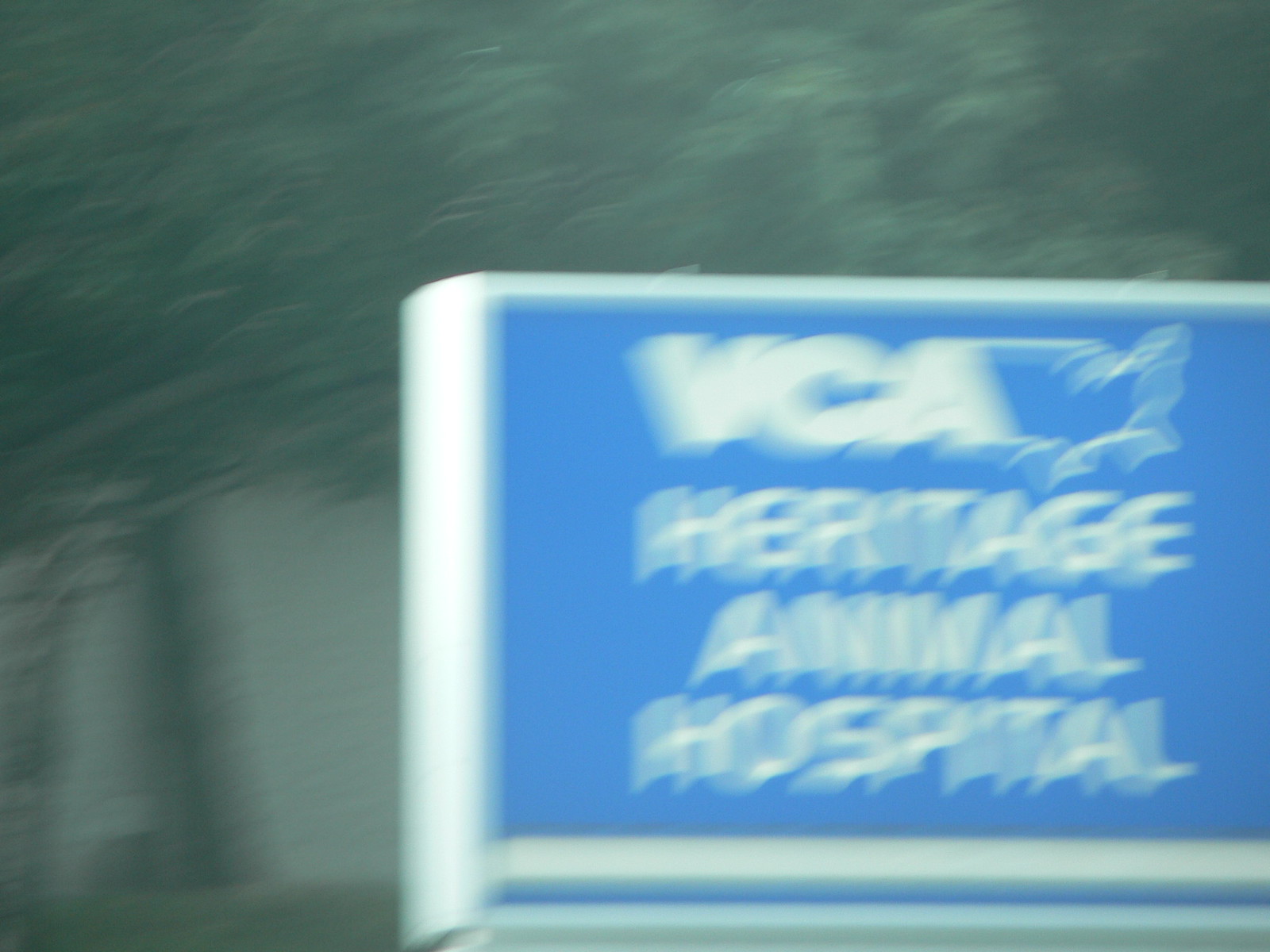This is a very blurry photograph of a business sign, specifically for an animal hospital. The sign is a blue rectangle with a white border and features white text. The main text reads "VCA" with a logo of the Continental USA next to it, followed by the words "Heritage Animal Hospital" beneath. In the background, there are trees, adding a greenish hue that almost resembles a watercolor due to the blur. The sign is positioned on the right side of the image, and it is daytime outside. The overall blurriness gives the letters a shadowy effect and obscures any other details or objects in the scene.